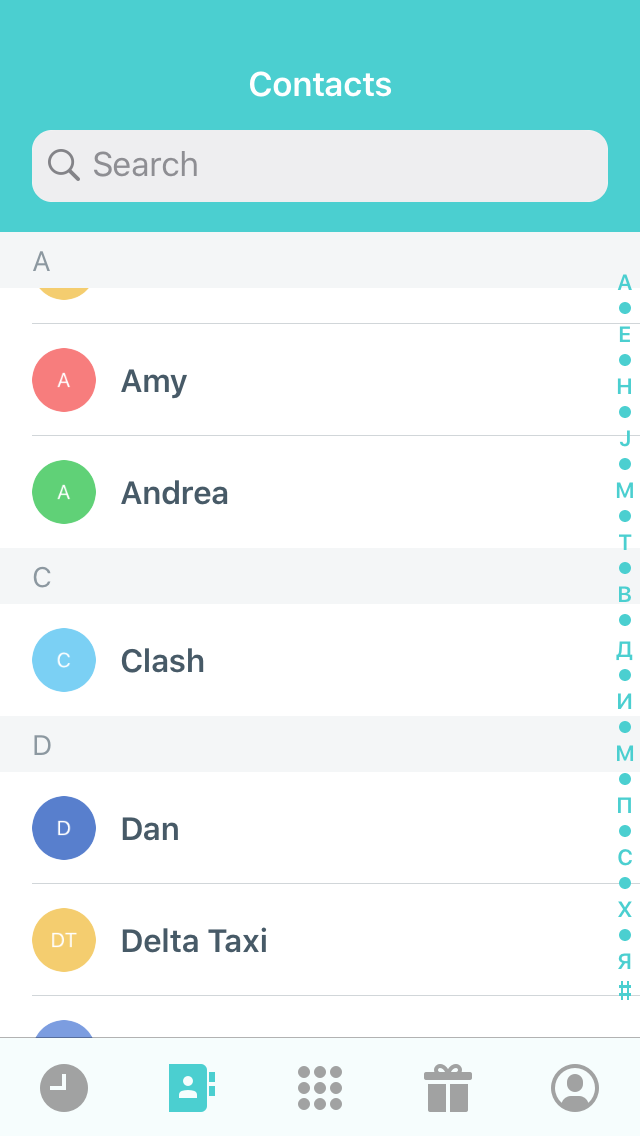The image appears to be a screenshot of the "Contacts" page on a cell phone, as indicated by the title "Contacts" displayed in white font at the top of the screen. Beneath this title is a blank search bar, labeled "Search" and featuring a small magnifying glass icon. 

The body of the image showcases a list of contacts organized in alphabetical order. The contacts are as follows:
1. Amy - represented by a red circle with a white "A" in the center.
2. Andrea - represented by a green circle with a white "A" in the center.
3. Clash - represented by a light blue circle with a white "C" in the center.
4. Dan - represented by a blue circle with a white "D" in the center.
5. Delta Taxi - represented by a light yellow circle with the white initials "DT" in the center.

Each colored circle representing the contacts features the respective initials prominently in the center, making the list visually organized and easy to navigate.